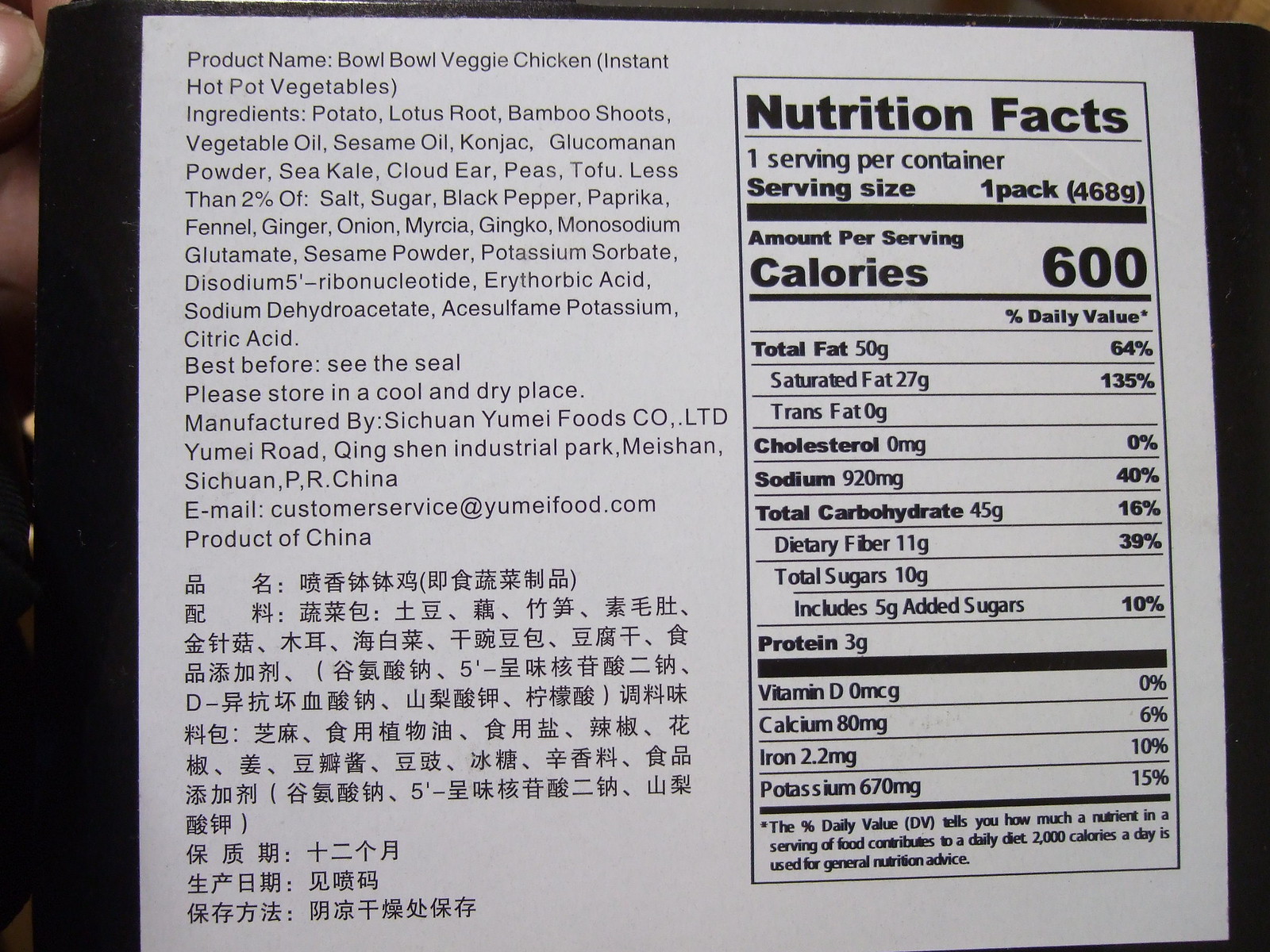The image showcases a portion of a nutrition label for a product named "Bowl Bowl Veggie Chicken Instant Hot Pot Vegetables". The top part of the label, including the full product name and brand, is not visible. The manufacturer is identified as Sichuan Yume Foods Co., indicating it is a product of China, which is further supported by the presence of Chinese characters below the manufacturer's information. On the right side of the label, the nutrition facts are prominently displayed, revealing that one pack contains 600 calories, with additional nutritional details provided underneath.